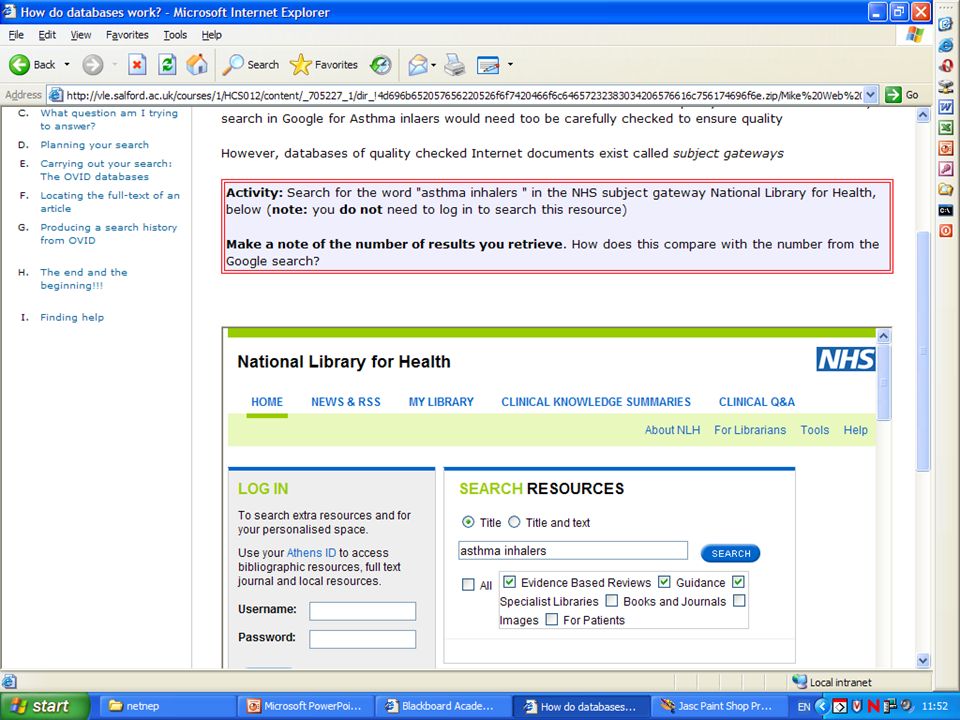The image features the homepage of a site provided by bla.salford.ac.uk, showcasing a variety of courses available for browsing. The user interface prominently displays a search result for "asthma inhalers," illustrating how users can obtain detailed information on specific topics. A panel titled "National Library for Health" is visible, offering options for logging in or using the search function without signing in. The search feature allows users to refine results by title, title and text, and includes evidence-based reviews, guidance, specialist libraries, books, and images. 

On the left-hand side of the page, a list of categorized options organized alphabetically—A, B, C, D, E—is present, enabling users to quickly navigate to areas of interest. Examples of these categories include "Planning Your Search," "Carrying Out Your Search," and "Locating the Full Text of the Article," among others. The detailed and intuitive layout of the homepage allows for a seamless search experience, catering to a wide range of informational needs.